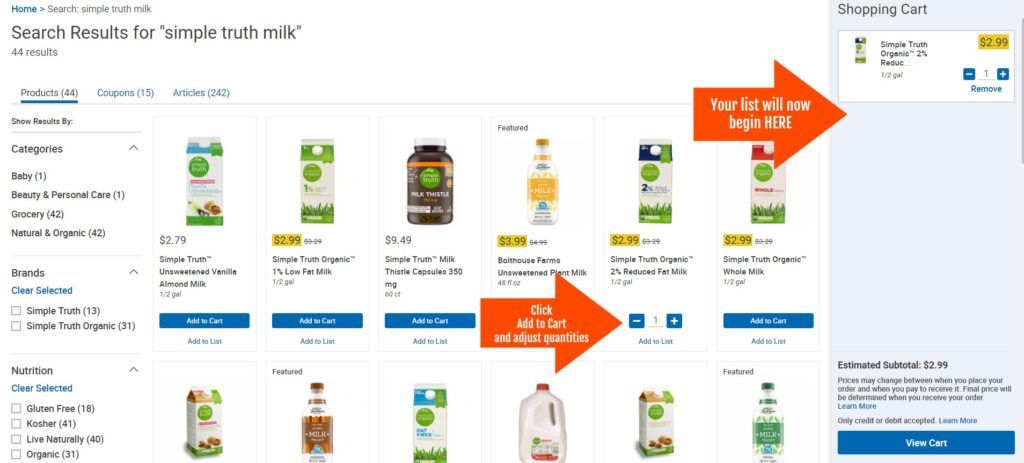The image depicts a webpage displaying the search results for "simple truth milk." In the top left corner, within quotation marks, it reads "search results for simple truth milk." Below this, there are three categories listed: "Products," "Coupons," and "Articles," with corresponding counts of search results shown next to each category. The "Products" category, which has 44 items, is currently selected, as indicated by a blue underline beneath it.

Beneath these categories, there are additional filters for "Categories" and "Brands," and at the bottom of this section is a filter for "Nutrition," offering several selectable options for each filter type.

To the right, six product listings are displayed prominently. Each product shows its price, product name, and two action buttons: a blue rectangle labeled "Add to Cart" and an "Add to List" button underneath. Four of these products have their prices highlighted in yellow, while two do not.

An orange arrow under the fourth product explains, "click add to cart and adjust quantities," pointing towards the fifth product. This fifth product includes a quantity adjustment option with a plus and minus sign.

Above the sixth product, there is a note stating "your list will now begin here," directing to the right-hand side of the screen, where a shopping cart icon shows one item inside it. Below this icon, the balance is displayed along with a green or blue rectangle labeled "View Cart."

At the very bottom of the middle section of the webpage, there are six more product listings visible but without any accompanying product information.